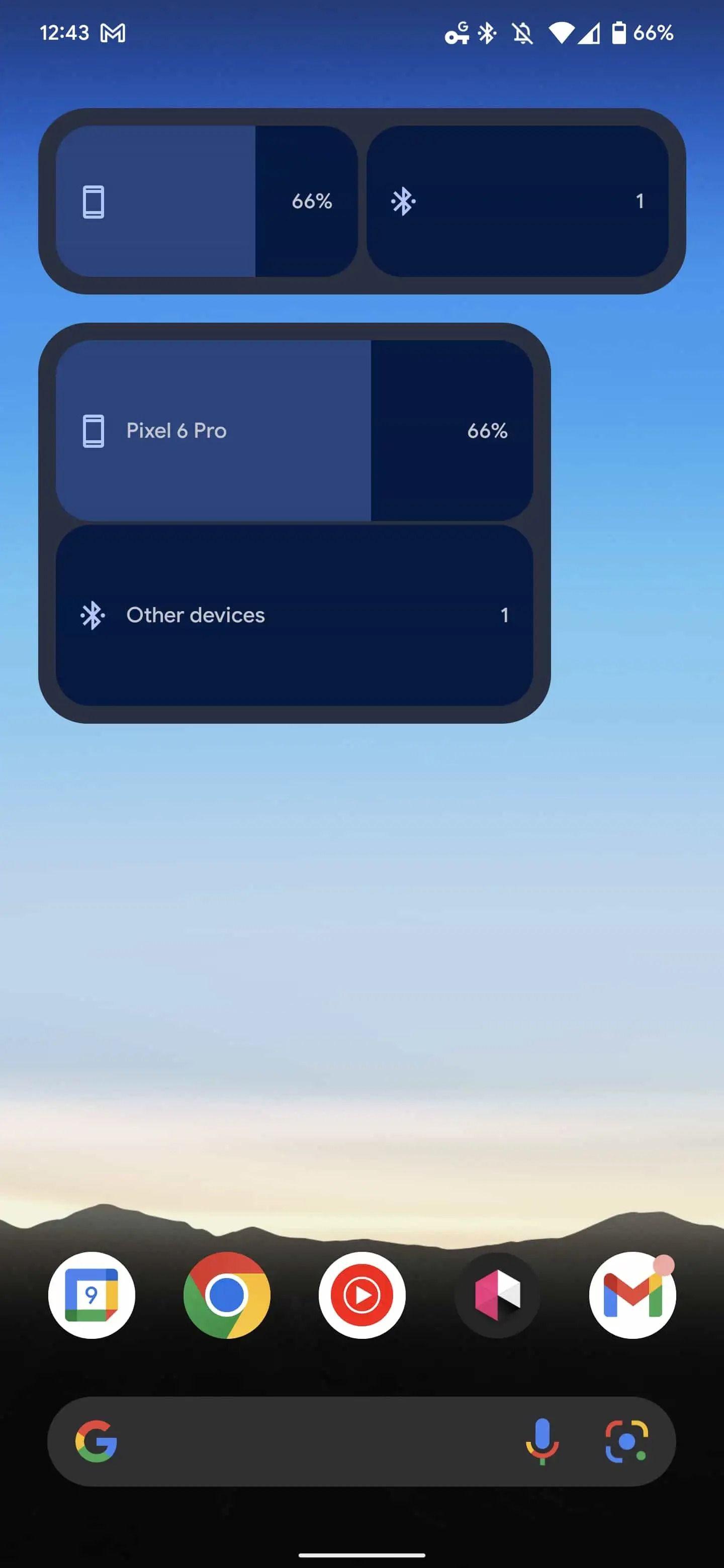This is a detailed description of a digital screenshot taken from a Pixel 6 Pro smartphone. The screenshot was captured at 12:43 PM, as indicated by the time at the top of the screen. The battery icon shows a charge level of 66%, and the Wi-Fi symbol is fully connected. The background image features a serene landscape with a mountain and a sky that suggests it is early evening.

On the home screen, various apps are visible. Prominently featured is the Google Chrome app with its distinctive red, green, yellow, and blue color scheme. Additionally, there is a Google search bar positioned on the screen, which includes a microphone icon for voice searches and a recognizable Google logo.